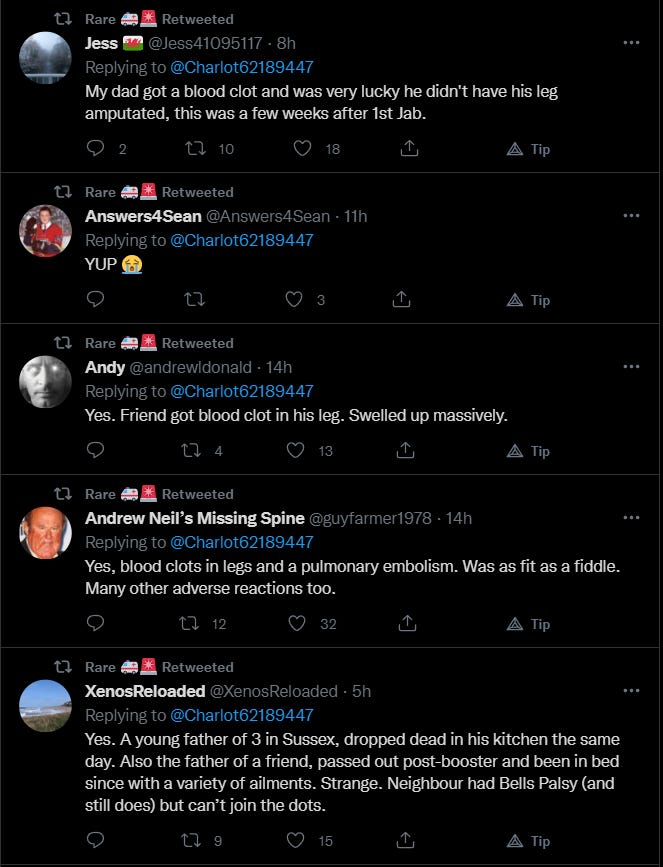The image showcases a segment of a Twitter feed displayed in dark mode, featuring a total of five posts. The background is black, and the text is in white, while usernames appear in blue. All posts are either replies or retweets addressing a user named @charlotte62189447, with each message relating to adverse reactions to vaccinations. 

1. Jess (@username) shares a personal account: "My dad got a blood clot and was very lucky he didn't have his leg amputated. This was a few weeks after the first jab."
2. Sean (@username) responds succinctly: "Yup."
3. Andy (@username) retweets with concern: "Yes, a friend got a blood clot in his leg, which swelled up massively."
4. Andrew Neal's Missing Spine (@username) details multiple reactions: "Yes, blood clots in legs and a pulmonary embolism; was as fit as a fiddle. Many other adverse reactions too."
5. Xenos Reloaded (@username) recounts several alarming incidents: "Yes, a young father of three in Sussex dropped dead in his kitchen the same day. Also, the father of a friend passed out post booster and has been in bed since with a variety of ailments. Strange. Neighbor had Bell's palsy and still does, but can't join the dots."

These posts collectively highlight various adverse reactions to vaccinations, contributing to a broader dialogue on the topic.